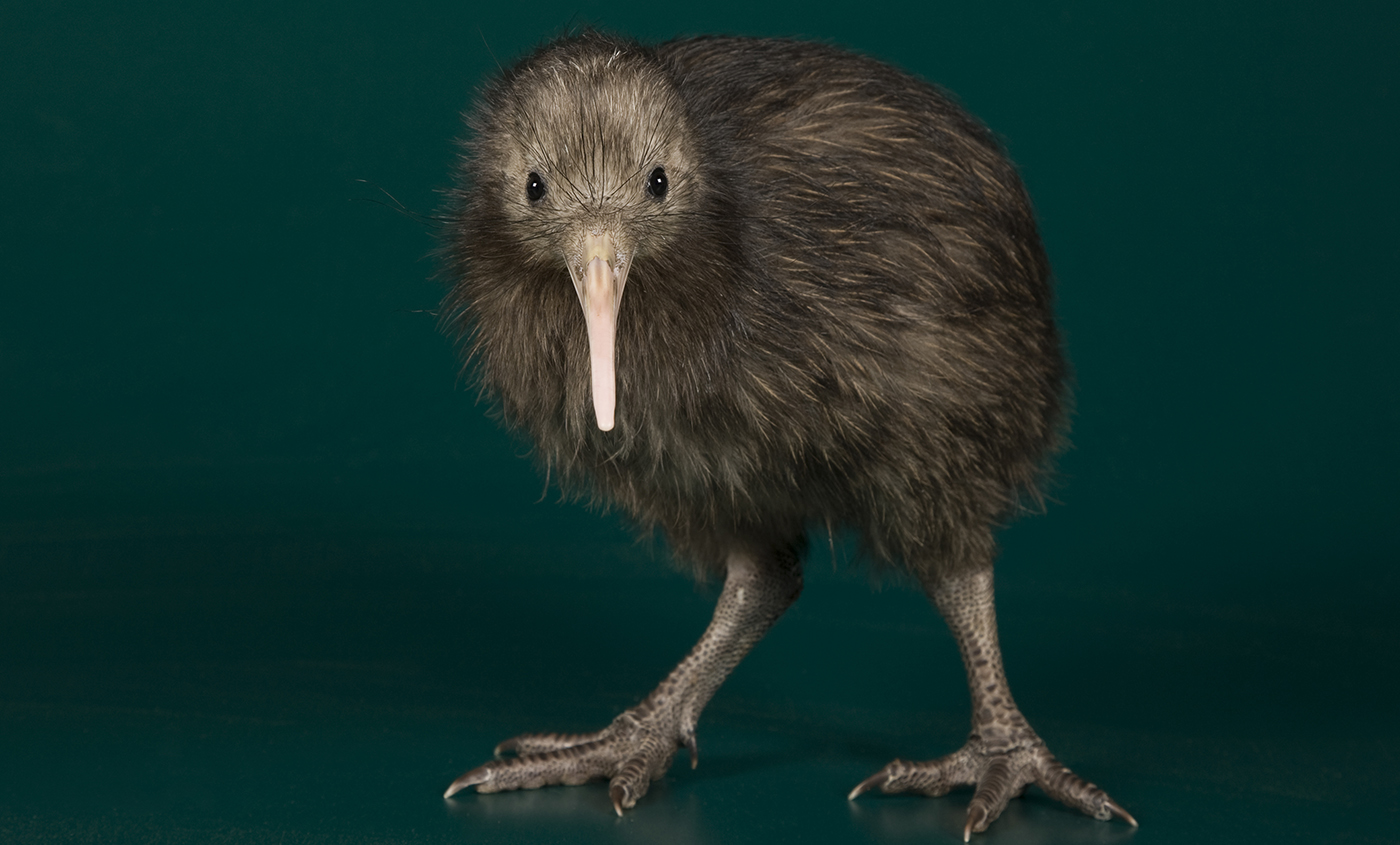The image features a kiwi-like bird standing on a digitally created abstract dark green background with a gradient effect, lightest behind the bird and darker along the edges. The bird, characterized by its dark brown, fur-like and slightly damp appearance, has no discernible wings or tail, highlighting its unique texture that resembles hair rather than feathers. It is positioned with its left side turned slightly towards the camera while its head, featuring black beady eyes and a medium-sized beak, faces directly towards the viewer. The bird's substantial back legs, reminiscent of dinosaur legs, are spread out, each with three toes ending in talons. The overall scene lacks additional objects or text, focusing solely on the bird, which may be either a real specimen or a highly realistic exhibit. The combination of light brown, brown, dark brown, tan, black, and dark green hues adds to the detailed rendering of the bird against its carefully created background.